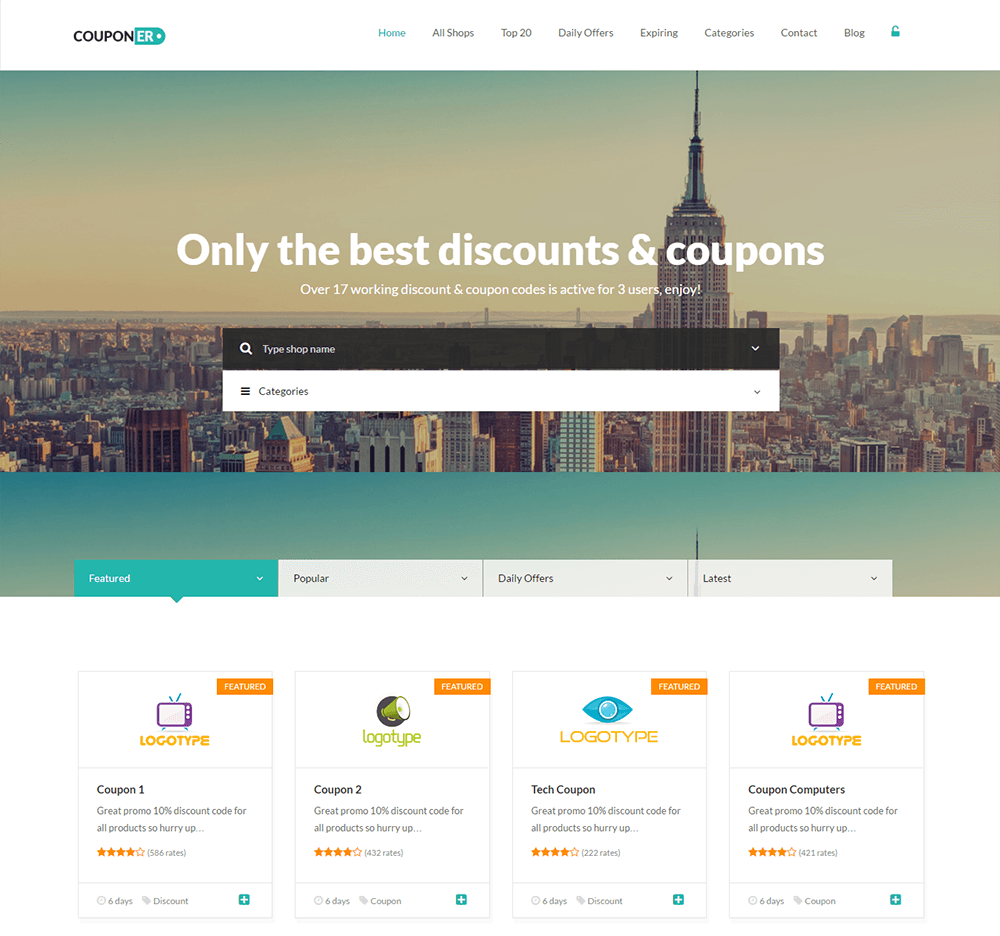The page appears to be designed for a travel company, but a closer look reveals it might be for a cashback or coupon site. The heading at the top reads "Coupon ER," and below it is a horizontally-oriented image of a cityscape dominated by a very tall tower. On the left side of the image, though the text is quite small and difficult to read, it states, "Only the best discounts and coupons. Over 17 working discount and coupon codes are active for 3 uses. Enjoy!"

Directly below the image, there's a black navigation bar featuring a drop-down menu where users can type in a shop name. Beneath this, there's a white bar labeled "Categories" with a downward-pointing arrow, indicating a selection menu for various categories.

The page is segmented into four sections, each represented by a different logo type. The first logo type seems to relate to electronic screens, the second likely pertains to household items, the third is marked by a blue eye, and the final one also seems to be related to screens. Each section includes user reviews, providing further insight and feedback on the available deals and categories.